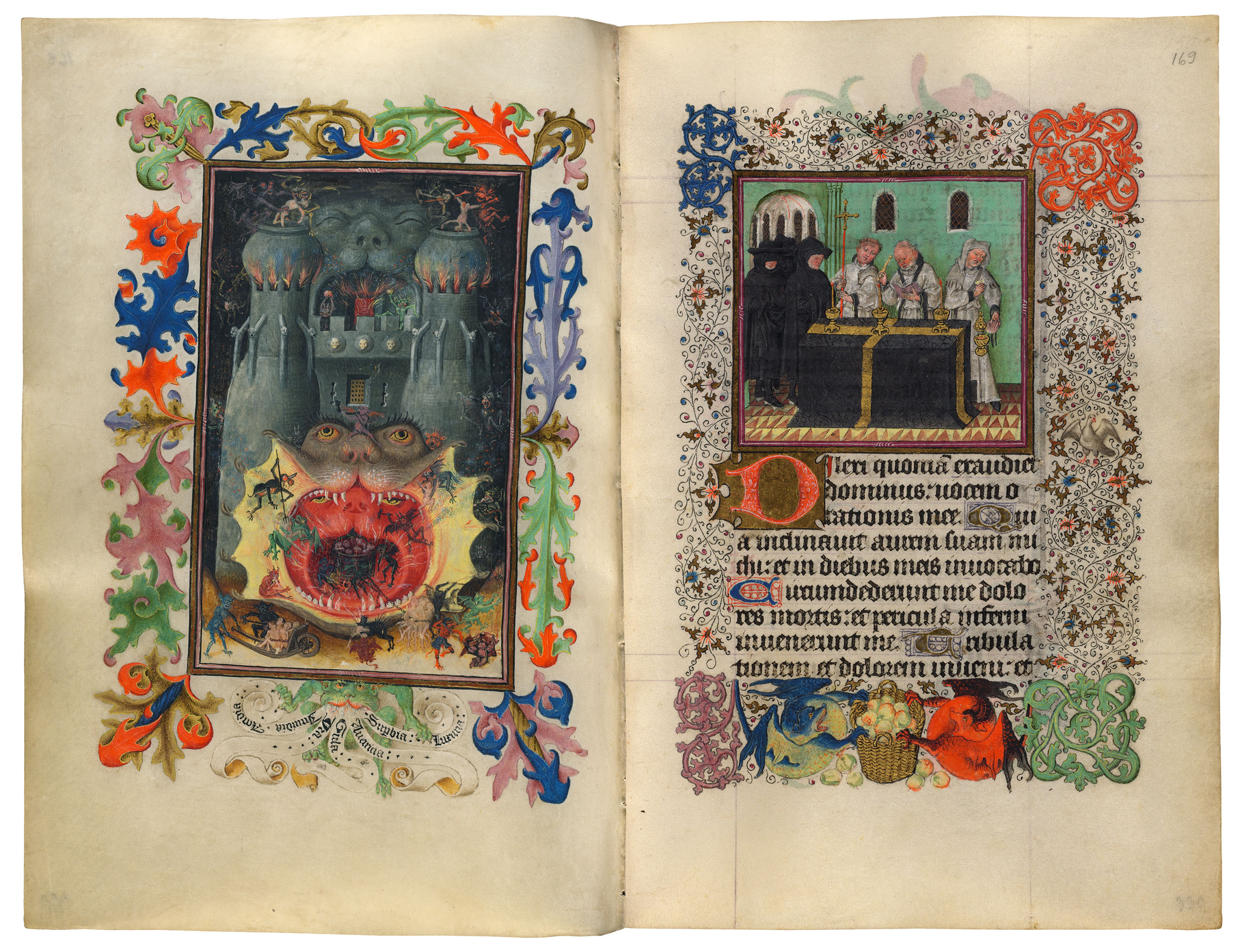This image depicts an ancient and meticulously crafted Bible. The tome appears aged, perhaps the kind of sacred text created by dedicated priests over the span of their lifetimes, each page inscribed with meticulous care and precision. On the left-hand side of the image, there is an elaborate illustration of a castle-like building, featuring two imposing towers—one on the left and one on the right. Dominating the center of this structure is a massive wooden drawbridge door, dramatically framed by the gaping mouth of a monstrous creature, offering a glimpse into its cavernous interior.

The right-hand side of the image portrays a group of priests gathered around a wooden table, deeply engrossed in discussion. Their expressions and gestures suggest the importance of their conversation, although the exact subject remains unknown due to the accompanying text, which is written in Latin—a language inaccessible to the casual observer. The overall composition speaks volumes about the rich history and profound reverence invested in this venerable religious manuscript.